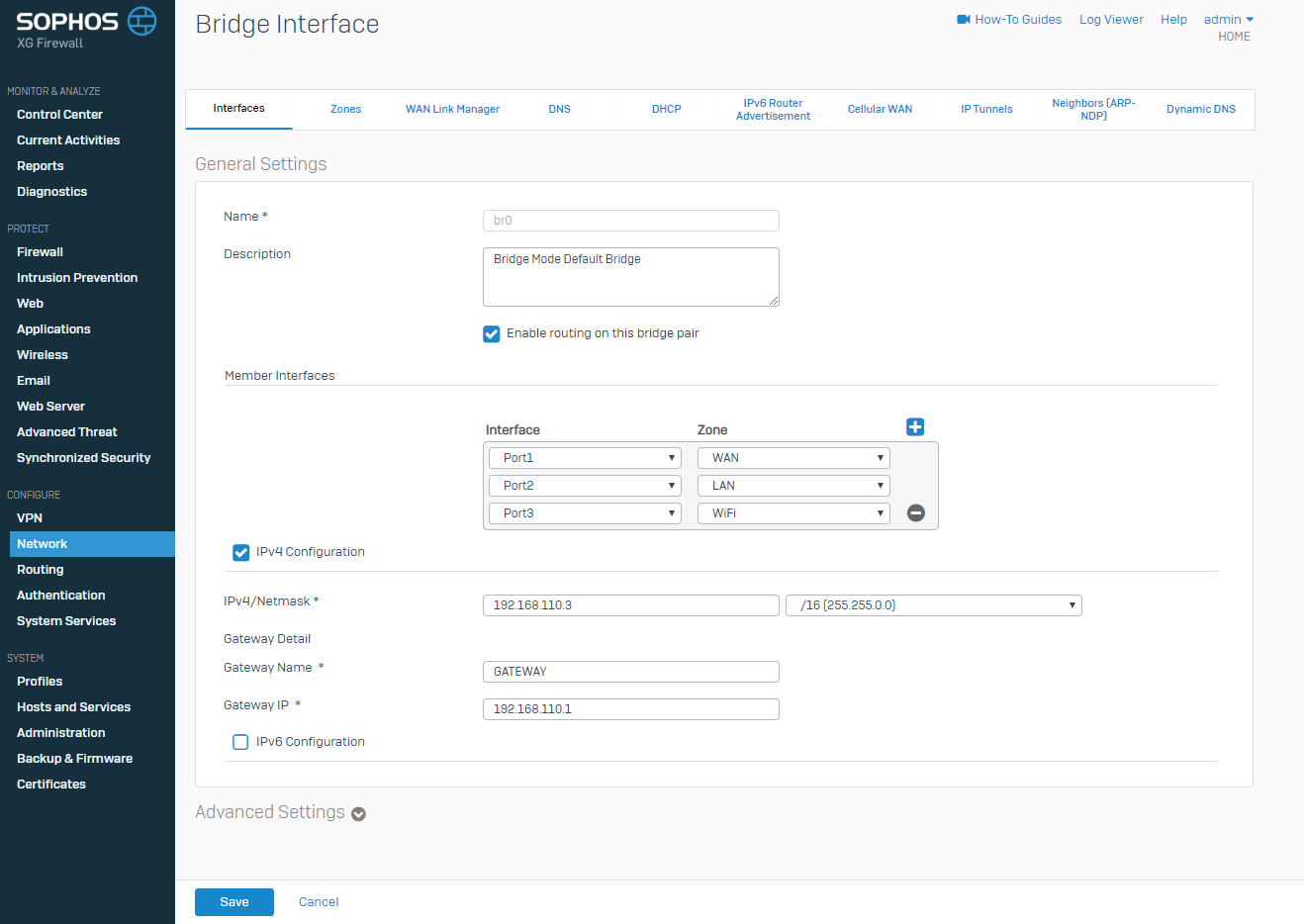The image is a screenshot featuring a user interface from Sophos, a cybersecurity company. The left side of the screenshot displays a vertical menu bar, which extends the entire height of the image. At the top of this bar, the word "SOPHOS" is prominently displayed in white, all-caps text. To the right of the text, there is a circular logo. Below the logo, a list of menu options in white text follows: "Contract Center," "Current Activities," "Report Us," and "Diagnostics," among others.

The main section on the right showcases a large, light-gray square. Positioned at the top left corner of this square, the text "Bridge Interface" is written in gray. On the right side of this header area, several blue menu options are visible. About five lines down from the top, there is a horizontal white rectangle serving as a header bar, beneath which is a gray space. A secondary large white square is positioned below this gray area, which seems to contain general settings.

In the general settings section, which is indicated by gray text reading "General Settings" on the left above the square, there is a settings window. This window is organized into two main sections: a list of controllable items on the left and corresponding drop-down boxes on the right. The first of these items is labeled "Name," followed by "Description" underneath, and "Member Interfaces" below that. The window further asks for network details, including fields for "Network," "Gateway Detail," "Gateway Name," and "Gateway IP."

This detailed layout suggests a sophisticated settings interface likely used for network configuration and management tasks.